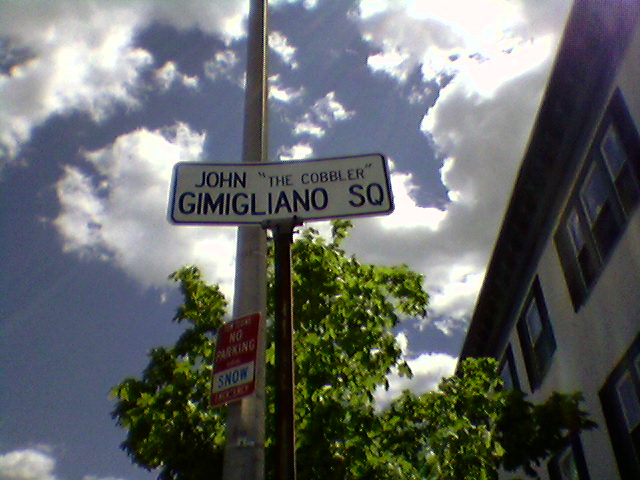This photograph captures the exterior of a building with a distinctive street sign prominently displayed in the center. The white, rectangular street sign features the text "John 'The Cobbler'" in black letters, suggesting it marks a street or perhaps a historical site. Below this text is "GIMIGLIANO SQ," further emphasizing its significance. 

To the right of the sign stands a charming black and white house, which appears to be at least two stories high and boasts numerous windows. The house exudes a pleasant and well-maintained appearance. Behind the street sign is a lush, bright green tree, adding a touch of nature to the urban scene. Also visible is a vertically rectangular "No Parking" sign with white letters on a red background. Below this sign, a white-bordered section with blue writing reads "Snow," indicating possible seasonal parking restrictions.

The background of the image features a vibrant blue sky, dotted with several large, fluffy white clouds, enhancing the overall picturesque quality of the scene.